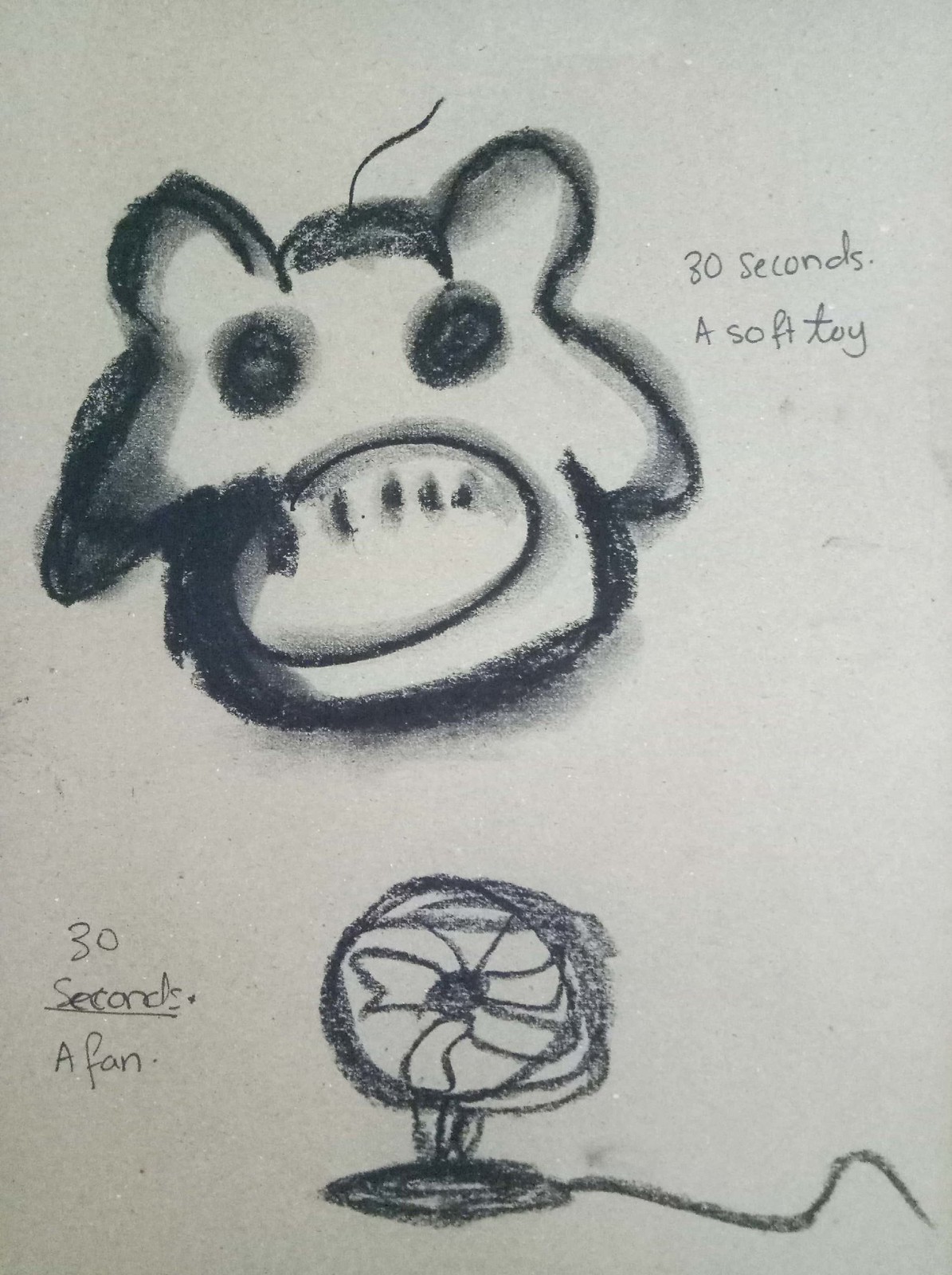The image features a pair of detailed sketches rendered in black ink on off-white paper. The top sketch depicts an animal resembling a pig, with a single strand of hair sprouting from its head and two prominent, round black eyes. The caption beside this drawing reads "30 seconds a soft toy," indicating the time taken to sketch it. Below this, there is another drawing of a table fan, complete with a cord trailing behind it. The fan's blades and structure are meticulously outlined, showcasing its characteristic round shape. To the left of the fan sketch, the caption reads "30 seconds a fan," also denoting the brief period used to capture this object. Both sketches are devoid of color, allowing the fine details and structure of the drawings to stand out against the plain background.